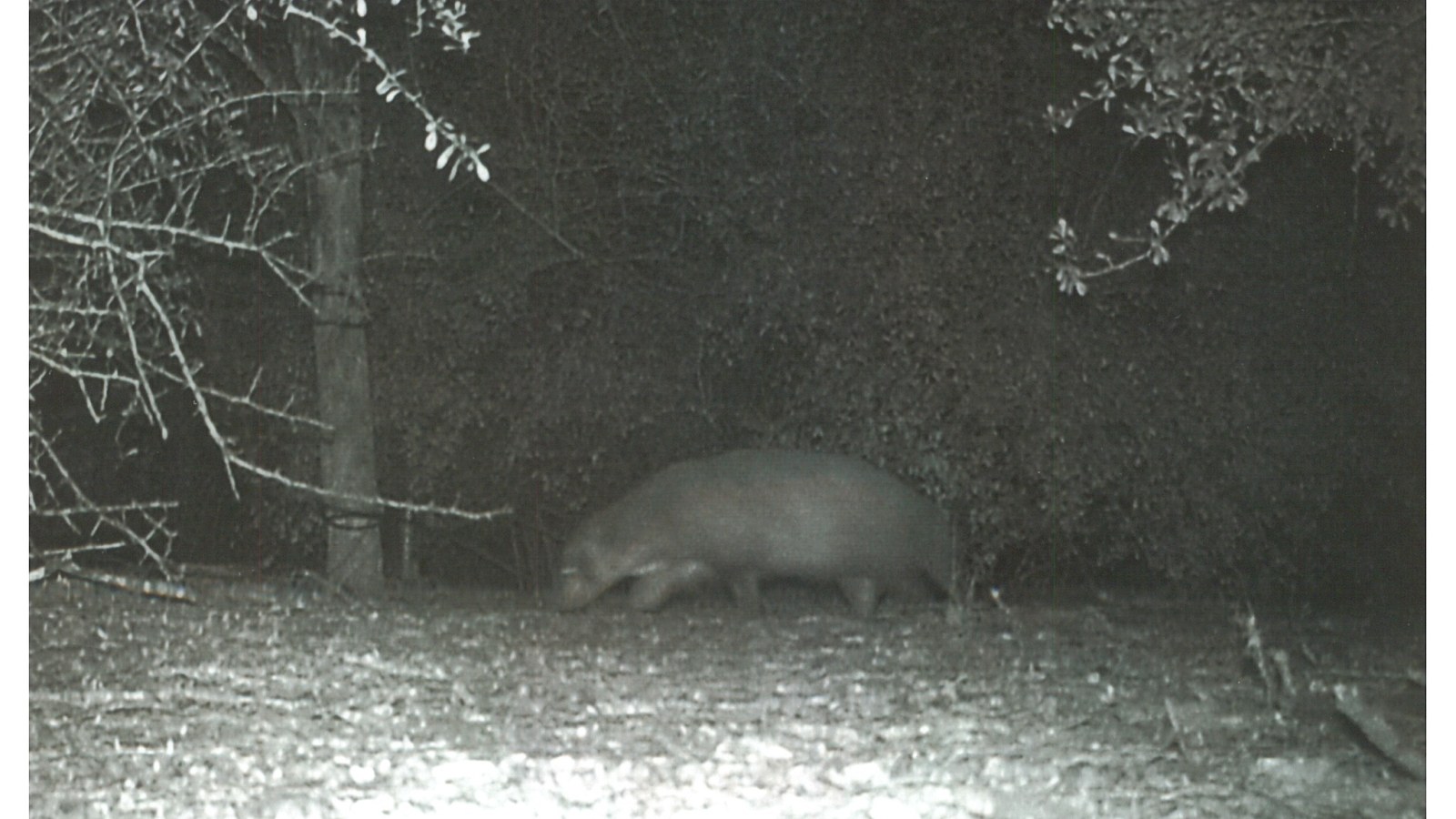This is a black-and-white, nighttime photograph likely taken using night-vision equipment or a trail camera, given the clarity and lighting of the scene. The central focus of the image is a large, indistinct animal, possibly a dog or a bear, positioned slightly toward the bottom center of the horizontal rectangle frame. The animal appears to be foraging or looking at the ground. Surrounding the animal, the setting is a dense outdoor environment with several trees and branches visible in the background and hanging from the top corners. The ground beneath the animal seems to be grassy with some dead branches strewn about. The overall scene is illuminated by a mysterious light source, enhancing the visibility of the animal and the surroundings amidst the dark, nighttime ambiance.